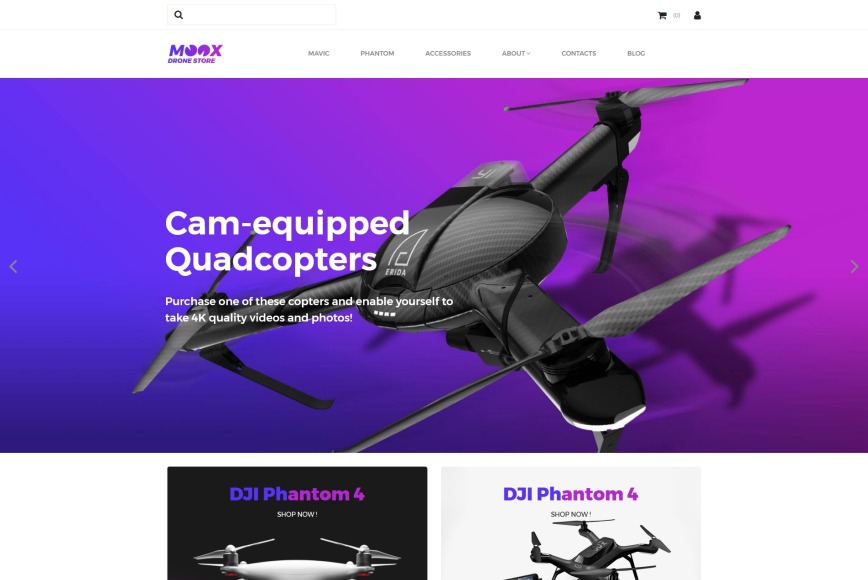This screenshot captures the upper left corner of a website prominently displaying the text "Monk's Drone Store" in vibrant purple font. To the right, the website menu features the options: Mavic, Phantom, Accessories, About, Contacts, and Blog. The background beneath this header transitions from purple to blue and showcases an illustration of a circular drone with three arms, each arm equipped with propellers. Overlaid on this background, in bold white text, is the phrase "Cam Equipped Quadcopters." Additionally, the text promotes the product, stating, "Purchase one of these copters and enable yourself to take 4K quality videos and photos." Below this promotional banner, there are two highlighted product boxes. On the left, a smaller black box features an image of a drone labeled "DJ-1 Phantom 4," accompanied by a "Shop Now" button. On the right, a contrasting white box showcases another drone, also labeled "DJ-1 Phantom 4," with a similar "Shop Now" prompt for easy access to the product.